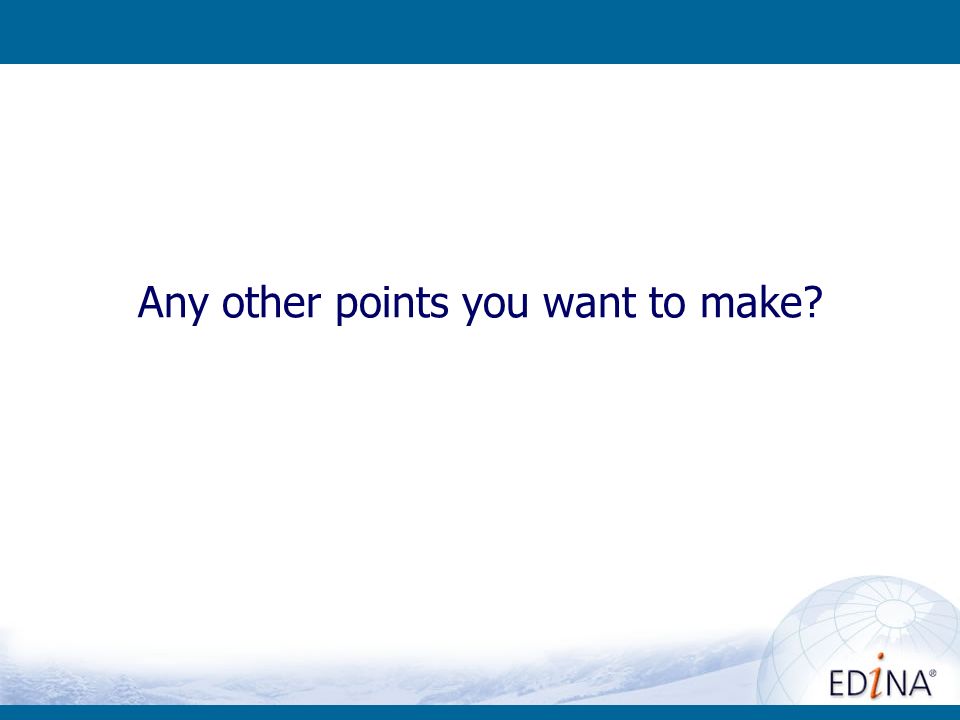The image predominantly features a white background with a narrow, dark blue band running along the top edge. At the center, the text "Any other points you want to make?" is displayed in the same dark blue color. The bottom part of the image has a very thin, dark blue line. In the bottom right corner, there's a partial, translucent globe in various shades of blue and white, with an orange detail. Overlaying the globe, the logo "ADINA" is written in blue letters with a lowercase orange "i." If you look closely, there's also a faint image of a mountain near the bottom of the globe. The simplicity of the slide contrasts with its detailed accents and text.